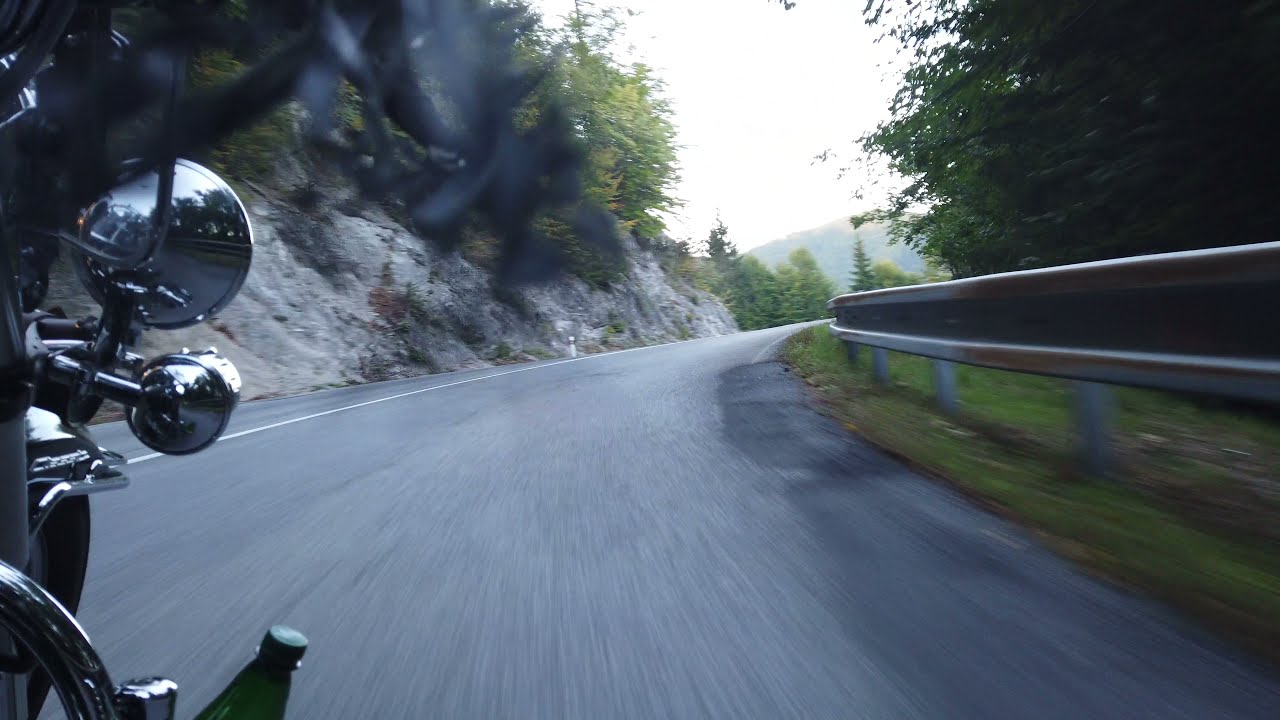The photograph appears to be taken from the perspective of a motorcycle rider using a dash cam or GoPro, mounted at eye level. The image is in landscape orientation, capturing a scene where the motorcycle dominates the left side of the foreground. The black motorcycle's handlebars, headlight, side mirrors, pedal, and possibly a water bottle are all partially visible, with motion blur evident, indicating the motorcycle is in motion.

The motorcycle is traveling on a wide, black asphalt road that narrows and curves sharply to the right in the middle ground. The left side of the roadway features a rocky, cliff-like hill adorned with green-leaved trees, adding a sense of rugged natural beauty. On the right side, a narrow grassy strip borders the road, accompanied by a low stone wall that mirrors the road’s curvature.

In the distance, the road leads to a horizon line where dense green trees and a misty mountain create a scenic backdrop. Above this landscape, the sky is overcast and washed out, contributing to a moody and dramatic atmosphere. In the upper right corner, beyond the stone wall, a dense grove of leafy green trees stands mostly in shadow, emphasizing the contrast between the shaded areas and the cloudy sky.

Motion blur is evident in the foreground, particularly on the road beneath the motorcycle, illustrating the bike’s forward movement. The overall composition combines the dynamic elements of a motorbike journey with the serene and rugged essence of the surrounding landscape.